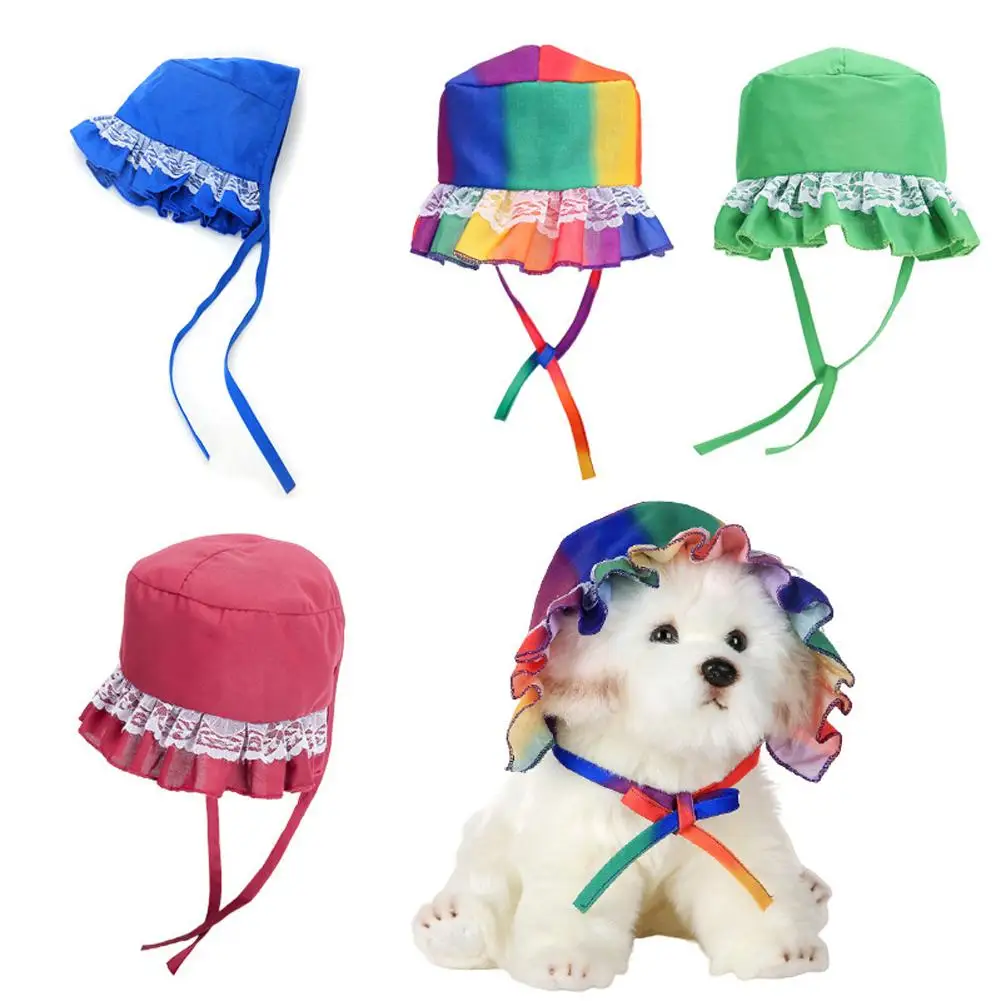This detailed image showcases a collection of five bonnet-style hats on a plain white background. In the upper left, there's a blue bonnet adorned with white lace and blue straps for tying under the chin. Next to it, in the center, is a vibrant rainbow-colored bonnet featuring colors like blue, green, yellow, red, purple, and orange, with matching rainbow straps. To the right of that, there's a green bonnet with white lace and green straps. The lower left corner has a pink bonnet with corresponding pink straps. Finally, in the lower right corner, a white stuffed toy dog is wearing the rainbow-colored bonnet, its straps tied securely around the dog's neck, illustrating how the bonnet would appear on a small toy dog.